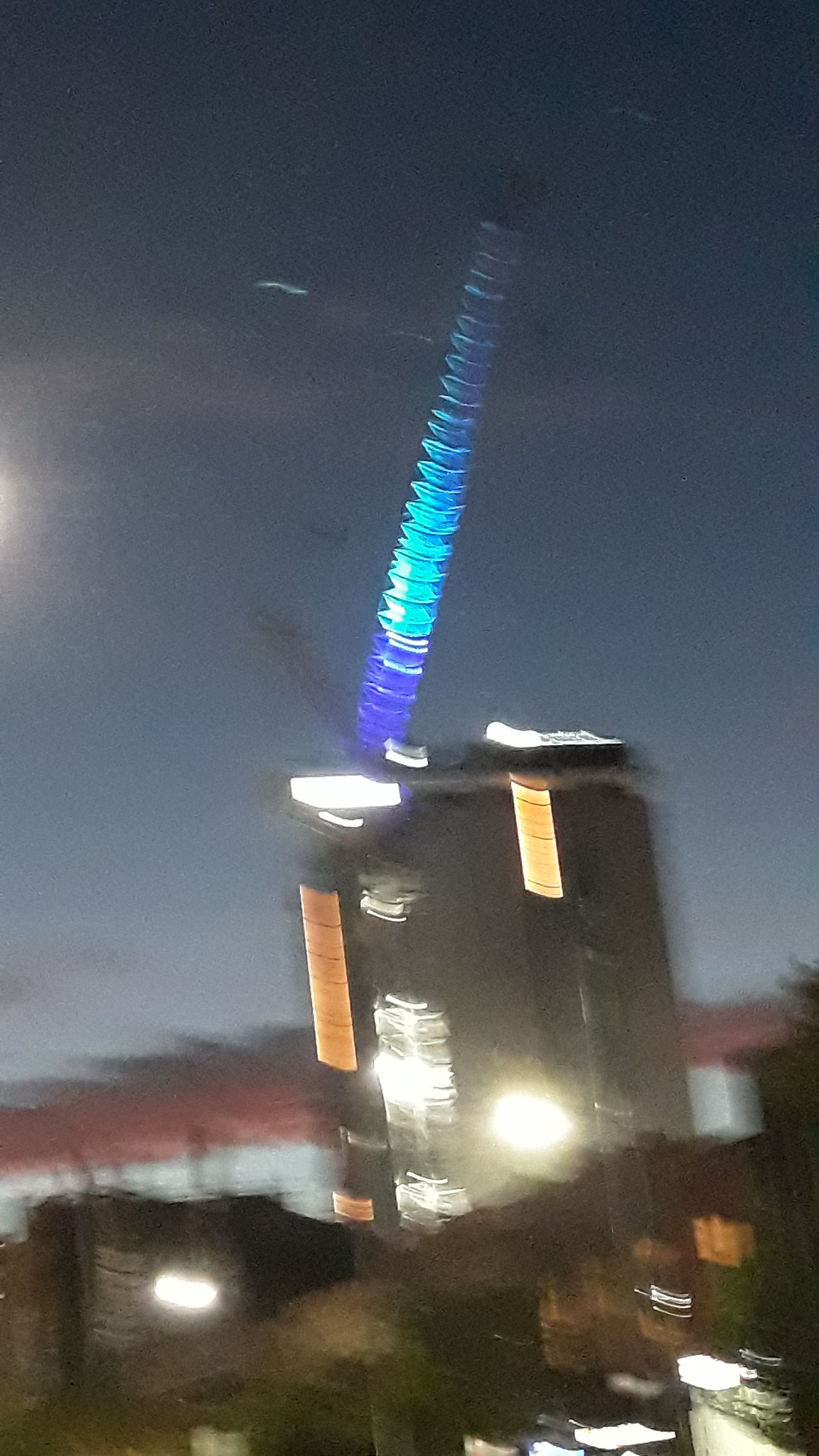A blurred photograph captures a building illuminated by lights, suggesting motion from the photographer. The main focus is a multi-lit structure, though its features are indistinct due to the overall blur. Above the building, a captivating stream of light spirals upwards in varying shades of blue, transitioning from dark blue to teal and back. The background sky hints at the presence of additional structures, also blurred. Light reflections are prominent throughout the image, adding to the sense of frenetic energy.